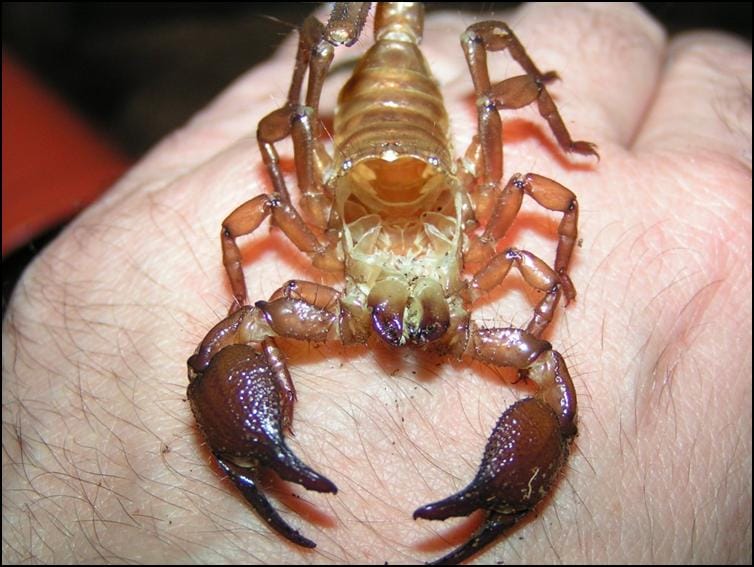The image showcases the back of a fair-skinned, hairy human hand, upon which lies a large, molted scorpion exoskeleton. The scorpion, primarily brown with darker brown claws, appears head-on with its top part cut open, revealing an internal white structure. The eight legs, lighter brown with a hint of red, splay out symmetrically from its body. The overall backdrop of the scene is indistinct but features a blurred mix of black and red hues. The hand, likely belonging to a Caucasian individual, complements the vivid detail of the scorpion molt.